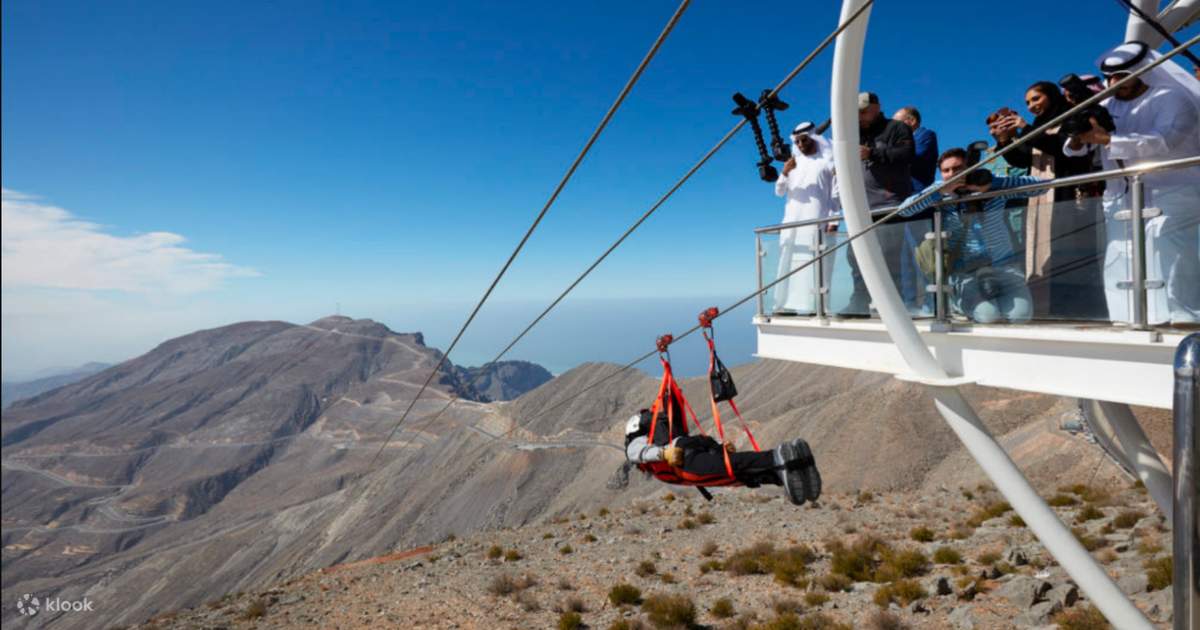The image captures an adventurous scene set against a stunning natural backdrop. A person, apparently strapped into an orange sling with two pulleys, is zooming down a zip line, positioned stomach down and face forward, wearing a helmet. This thrilling ride seems to descend from a high vantage point marked by a tall white tower situated to the right of the scene. The tower, featuring a glass railing, is crowded with people, many of whom are dressed in traditional Arabic clothing, suggesting a Middle Eastern location, possibly Saudi Arabia. These spectators, some holding cameras, appear to be capturing the moment. The background reveals a rugged, desert-like landscape with scrubby, dry mountains and a ridge stretching from left to right. The sky above is a lovely blue, dotted with a few clouds, adding to the overall beauty of this adventurous setting.